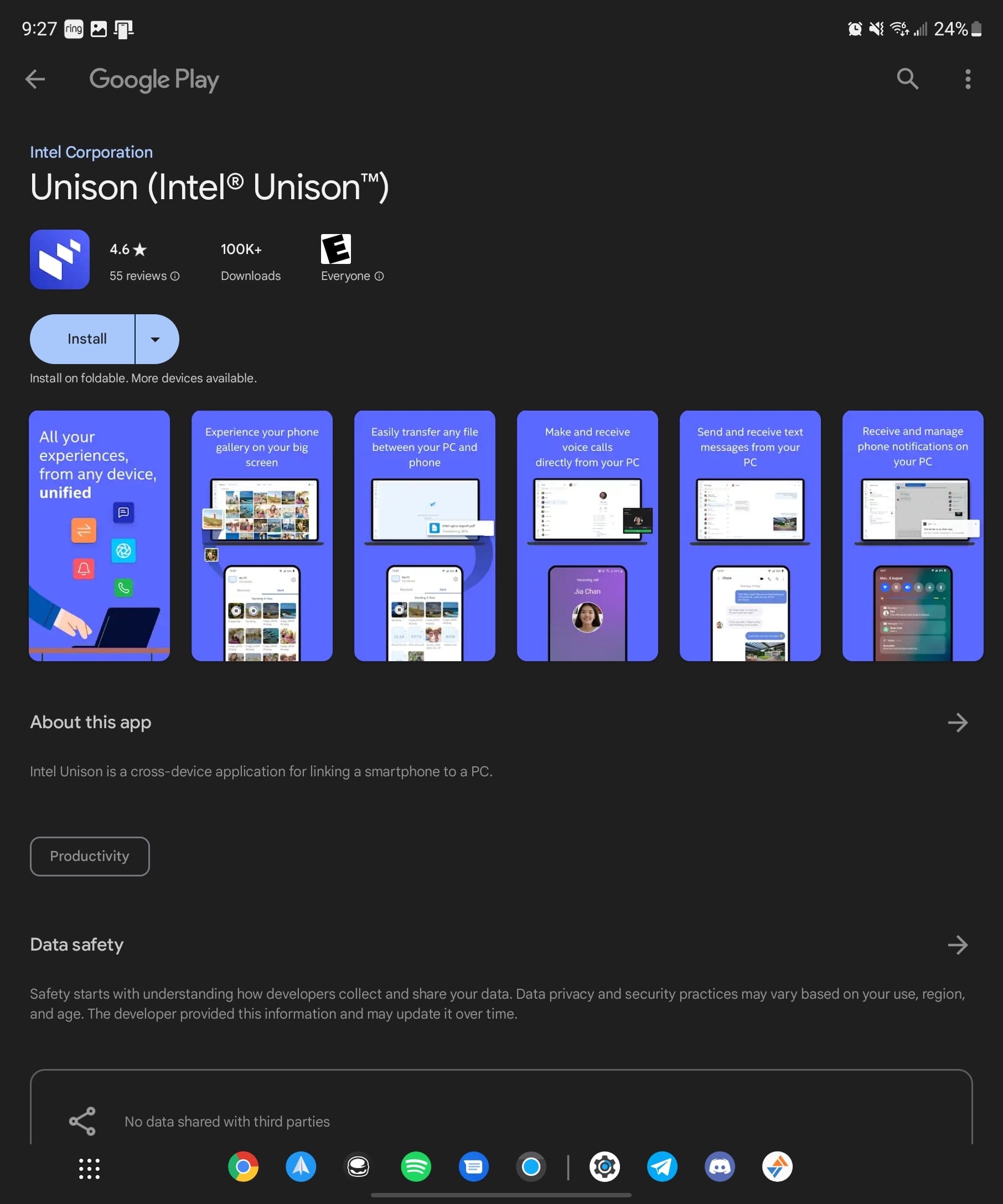This image depicts a screenshot from the Google Play Store app interface. At the top of the screen, prominently on the left side, the text "Google Play" is displayed. Adjacent to this text is a back button, enabling navigation to the previous page. On the right side of the top bar, there is a search button, characterized by a magnifying glass icon, and a menu button, represented by three vertically stacked dots which likely provide additional options.

The highlighted app in the screenshot appears to be offered by Intel Corporation, as indicated by the light blue text beneath the Google Play logo. The app is named "Intel Unison," with "Intel Unison" enclosed in parentheses for emphasis. The app's icon features a dark blue square with three white screens arranged in it.

To the right of the app icon, the app's details are presented: a rating of 4.6 stars based on 55 reviews. Furthermore, the information reveals that the app has been downloaded over 100,000 times. The layout and details vividly indicate key information about the Intel Unison app's popularity and user reception on the Google Play Store.